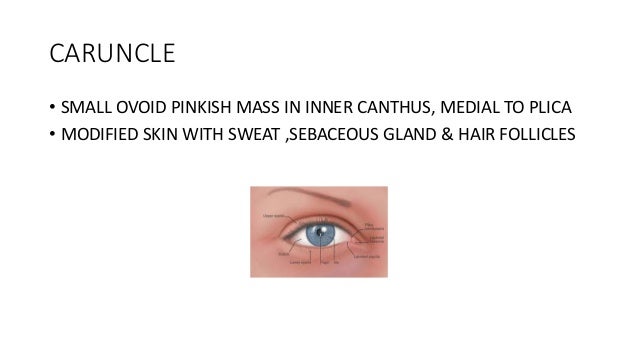The image is an educational slide focused on the eye, specifically a part labeled "CARUNCLE." The slide has an all-white background with three lines of black text at the top, running from left to right. The text reads "CARUNCLE" in capital letters, followed by two bullet points. The first bullet point states, "SMALL OVOID PINKISH MASS IN INNER CANTHUS, MEDIAL TO PLICA," and the second bullet point reads, "MODIFIED SKIN WITH SWEAT, SEBACEOUS GLAND AND HAIR FOLLICLES." Below the text is a small, postage stamp-sized image of a blue-eyed Caucasian woman's face, showing just a portion of her eye. The eye is directed straight ahead, and there are several tiny arrows and labels pointing to different parts of the eye; however, the labels are too small to be legible. The overall layout is simple, with the image centered beneath the descriptive text.